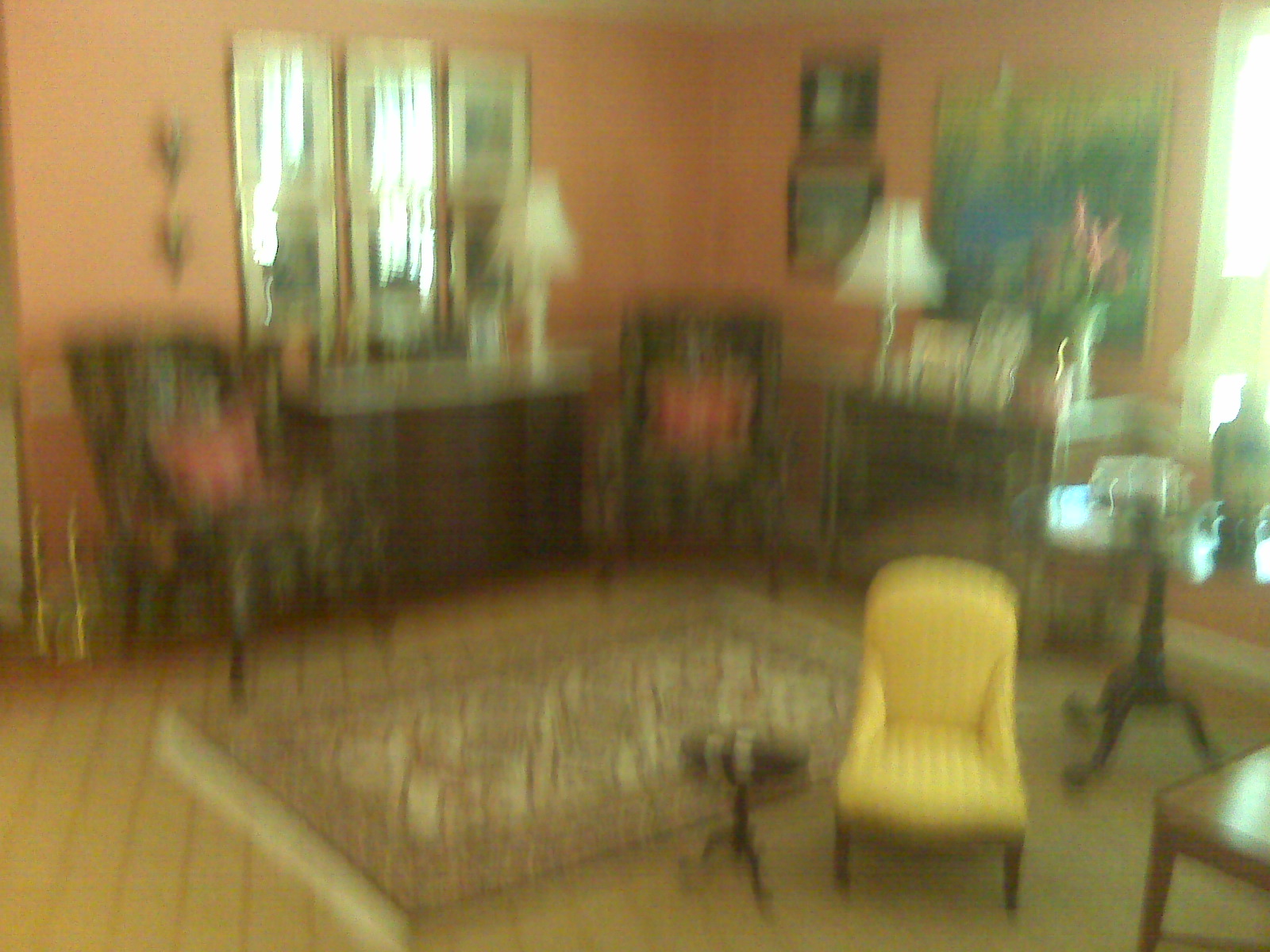The photograph depicts an outrageously blurry image of what seems to be a Victorian-esque room. The floor features a pale yellow carpet adorned with diagonal brown stripes or possibly a diamond pattern, complemented by a central Turkish rug in shades of cream, brown, and hints of red. Dominating the foreground is a pretty yellow chair paired with a three-legged Victorian side table. In the background, two matching floral print chairs with pale pink pillows are positioned, likely under a window that allows some light to seep into the room. The peach or pink-colored walls in the background host various artworks, possibly including nature scenes, flanked by two mirrors. Across from the seating arrangement is a buffet that appears to have a marble top. Each surface, whether a table or the buffet, features a lamp, contributing to the room's warmly lit ambiance. Despite the blurred quality, the scene showcases a richly detailed and decorated space that blends comfort with classical elements.